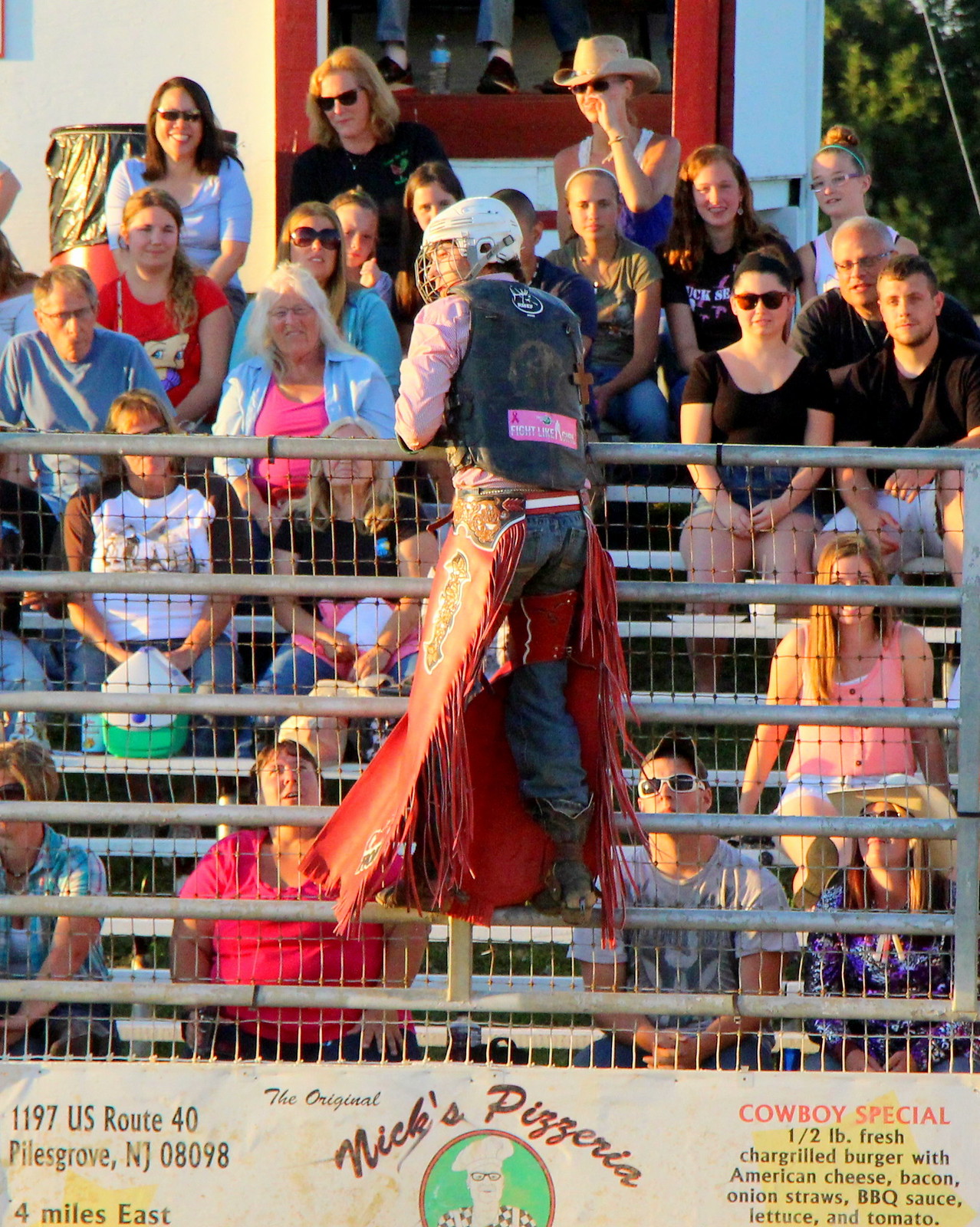This detailed photograph captures a thrilling moment at a rodeo event in Powells Grove, New Jersey. Central to the image is a rodeo participant, likely a bull rider, who has climbed up a metal fence, perhaps to evade a bull. He is seen wearing a distinctive rodeo outfit: a white helmet with a face guard, a pink shirt, a black protective vest, blue jeans, and brown boots. Additionally, he has a red skirt-like garment typical of rodeo costumes. His back faces the camera while his head turns to the left, allowing for a glimpse of his determined expression.

The fence he is clinging to features an advertisement for "Nick's Pizzeria," proudly displaying a friendly chef's illustration and promoting the "Cowboy Special." The stands behind the fence are packed with spectators, arranged in at least seven or eight rows. The crowd, a mix of smiling men and women, is attentively watching the spectacle unfold under the sunny sky. The arena’s vibrant atmosphere adds to the excitement, highlighting the shared enjoyment of this traditional cowboy event.